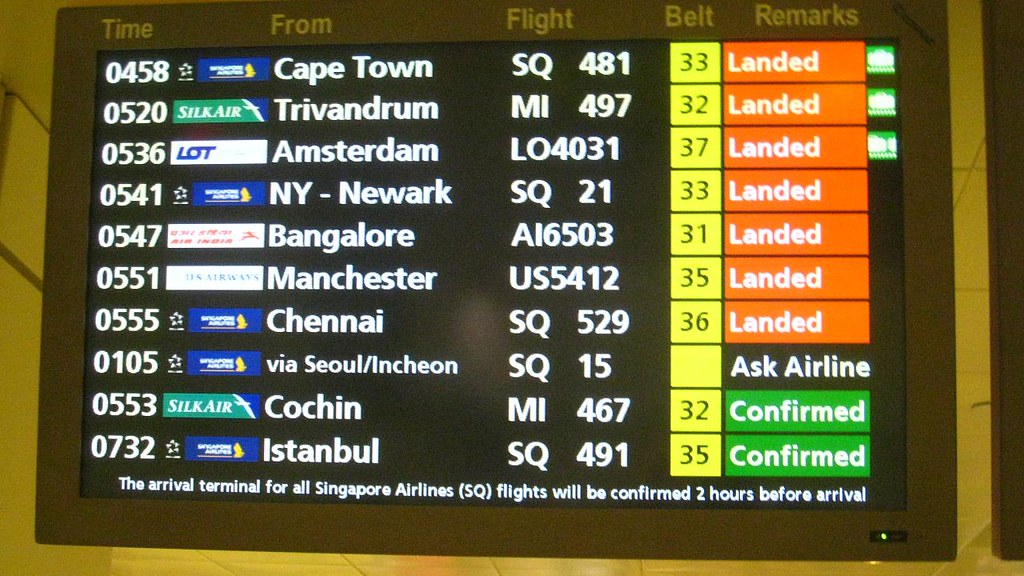The image depicts a close-up of an airport information screen displaying a detailed list of flight arrivals. The screen is organized into multiple columns: the first column indicates the time of arrival, followed by the origin of each flight (e.g., Cape Town, Trivandrum, Amsterdam, New York-Newark, Bangalore, Manchester, Chennai, Seoul-Incheon, Köln, Cochin, and Istanbul). There's also a column for flight numbers and another for remarks on their status. Most notably, flights that have landed are marked with a red border and the label "landed" in white text. There is one flight with the remark "Ask Airline," and two flights at the bottom have a green background with the status "Confirmed." Additionally, some airlines have stars or green symbols next to them, though their significance is unclear. Notably, at the bottom of the screen, white text reads, "The arrival terminal for all Singapore Airlines flights will be confirmed two hours before arrival."